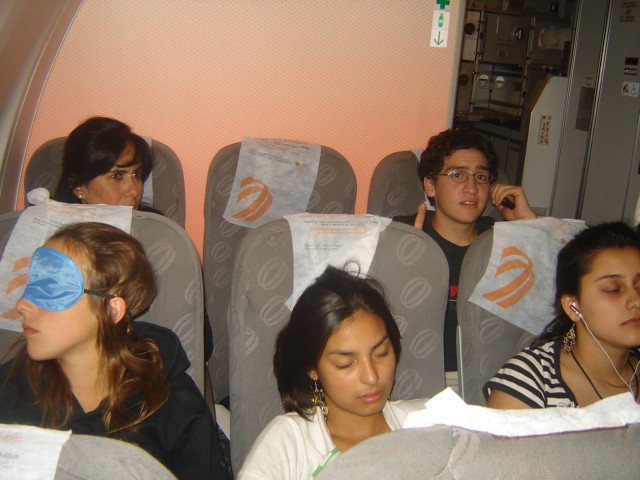The photograph captures a group of people resting on an airplane, clearly indicated by the white sanitary barriers on the backs of the gray seats. There are five individuals seated across two rows in this image. In the front row, three women are sleeping: the woman on the left wears a black jacket and a bright blue eye mask; the middle woman in a white dress appears to be fast asleep; and the woman on the right, dressed in a black and white striped t-shirt, has earphones in. Behind them, in the back row, the left seat is occupied by a teenage boy wearing glasses, while the middle seat remains empty. On the right, an older woman, possibly in her 40s, sits by the window with the plane's light coral walls in the background. The photograph also hints at a grey-colored shelf on the right side of the frame.